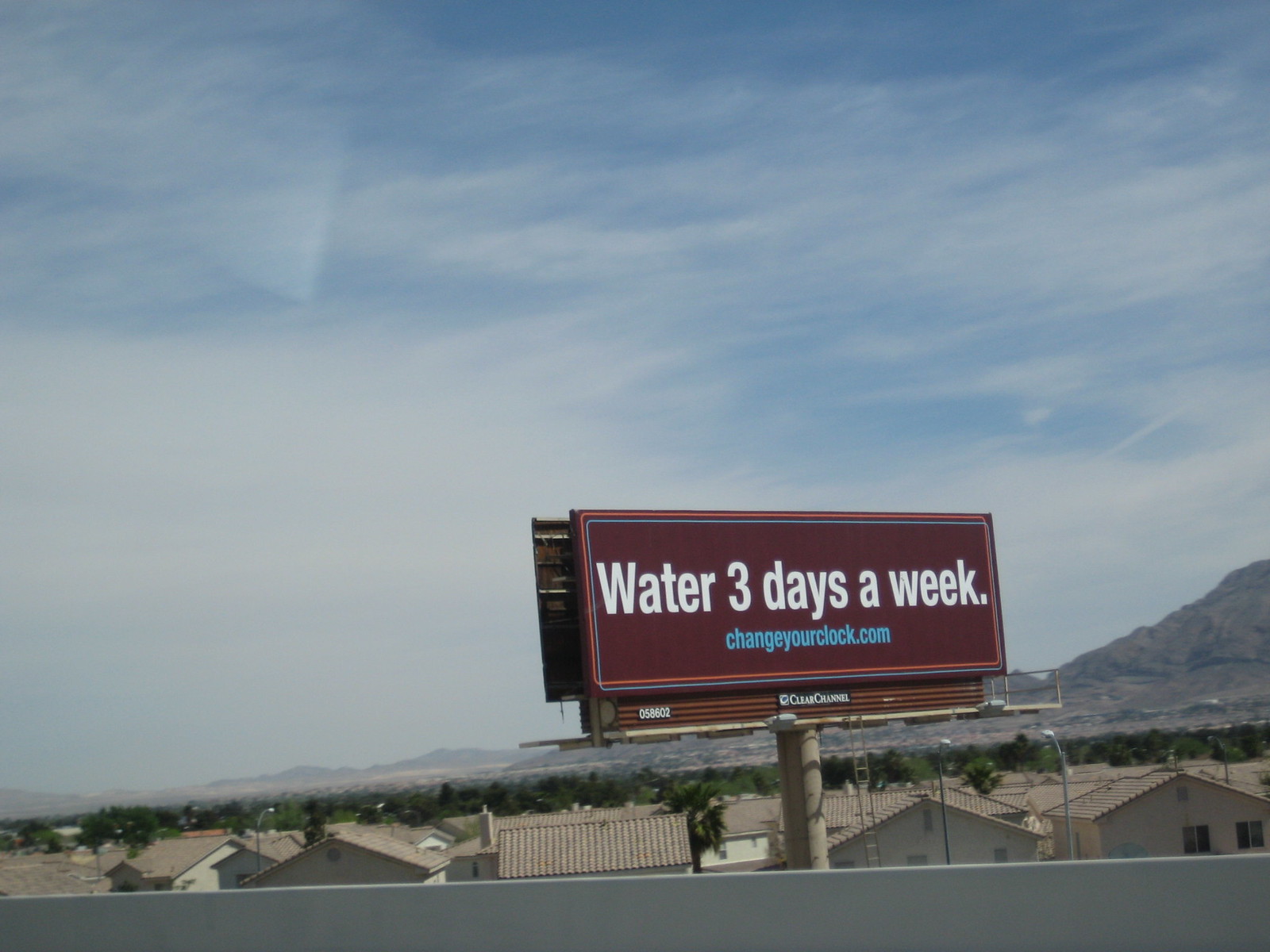Captured from an elevated vantage point, this image prominently features a dark maroon or brownish billboard with a red and blue border. Centrally displayed on the billboard, in large white text, are the words "Water 3 days a week," with the smaller blue text "changeyourclock.com" situated below. The billboard is owned by Clear Channel, identifiable by the company’s name and serial number 058602 displayed at the bottom. The scene encompasses a sprawling residential area characterized by white buildings with tan or light brown metal roofs. In the background, low-spread mountains provide a natural backdrop, while the sky above is dotted with thin, wispy clouds against a blue horizon. The suburban landscape below suggests a possible location within regions such as California or Arizona.